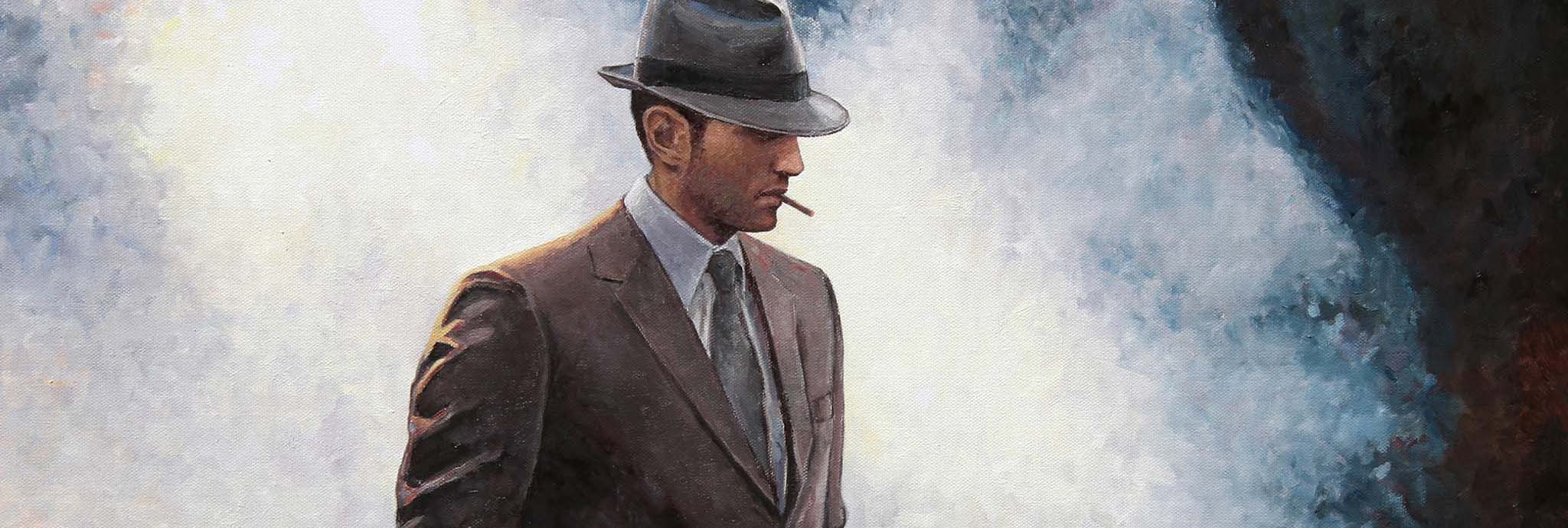In this horizontal color image, possibly a stylistic drawing or painting, we see a close-up of a Caucasian man from head to mid-chest, wearing a light gray fedora hat with a black band around its base. His fairly pale skin, despite a tan, contrasts with his serious, almost neutral expression. The brim of the hat casts a shadow, slightly obscuring his eyes as he looks off to the left and somewhat downward. He has brown hair and a single cigarette or cigarillo between his lips. He is dressed in a brown suit jacket, paired with a white collared shirt and a black tie. The background is abstract, blending white and yellow cloud-like hues on the left with a darker navy blue or black on the right, creating a dramatic contrast. The light source appears to be behind him, illuminating his shoulders while leaving the front of his body in shadow.